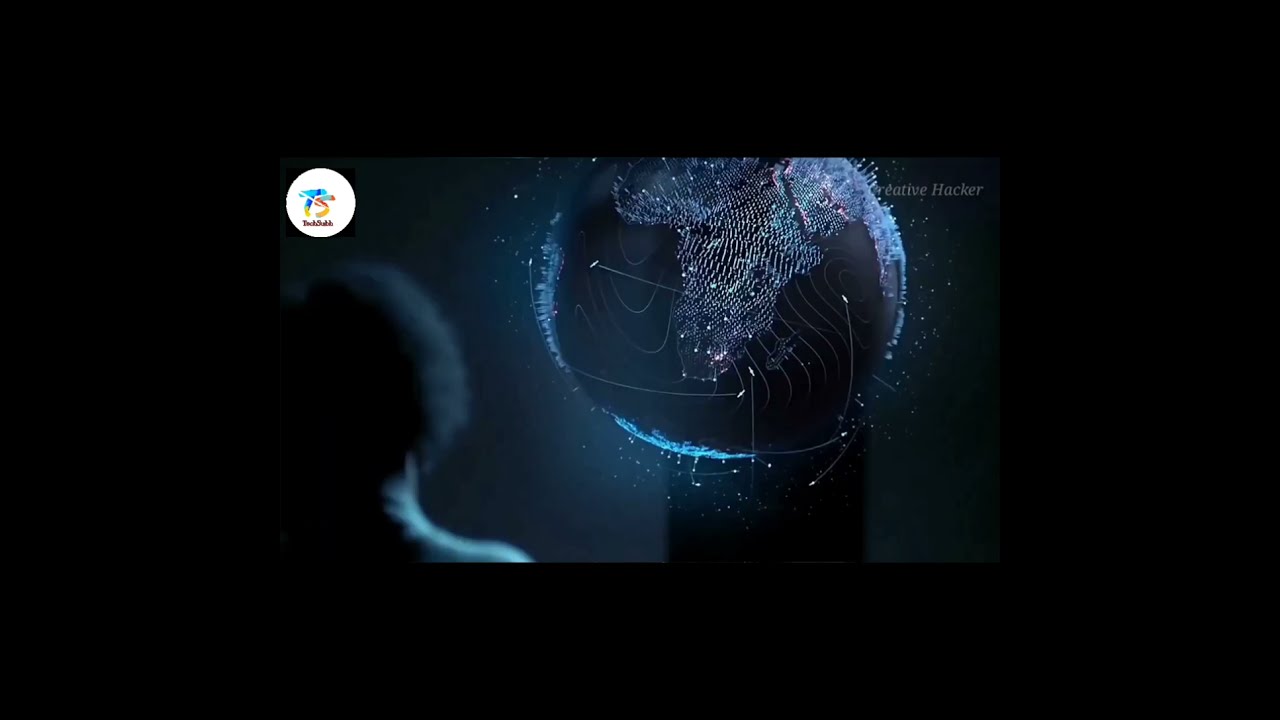In this captivating image, set against a dark, outer space-inspired background adorned with glittery white sparkles, a glowing black globe takes center stage. This suspended globe illuminates the various land masses with a striking blue light, while the water areas remain black. The intricate 3D elements of the globe, including raised portions, highlight different countries and cities, adding to its digital, high-tech aesthetic. Positioned at the lower left, a person with bushy, curly hair wearing a light-colored shirt stands with their back to the camera, gazing at the globe. In the upper left corner, a white circle logo with the letters "TS" or "T5" in blue and yellow is prominently visible. Meanwhile, the upper right corner features the text "creative hacker." The image, filled with sparkles and digital effects, evokes the feel of a tech-related news article, possibly one discussing cybersecurity or hacker organizations. Fairy dust-like particles further enhance the mystical atmosphere of this visually compelling scene.